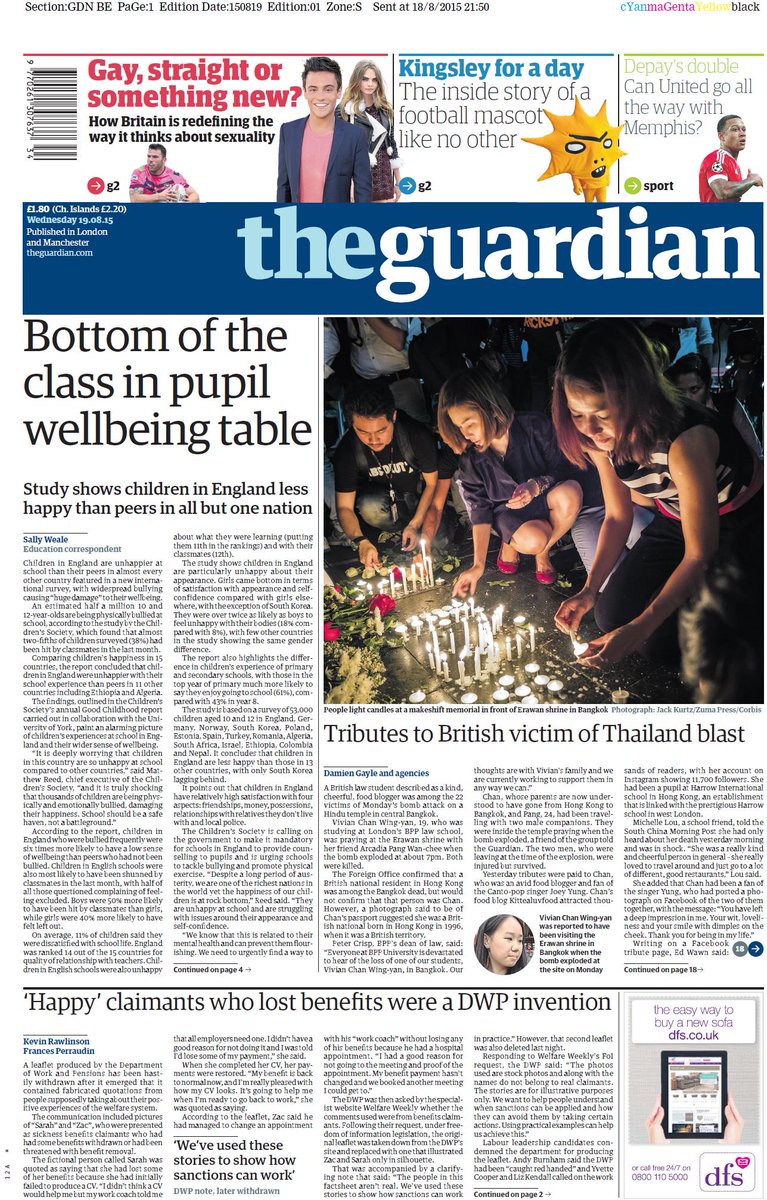This is a screenshot of the front page of The Guardian's online newspaper, dated August 18th, 2015. The publication's name, "The Guardian", is prominently displayed in a large, bold blue bar across the top of the page. This UK-based publication's front page features a central image depicting three young individuals lighting candles at what appears to be a memorial. The headline beneath this poignant photograph reads, "Tributes to British Victim of Thailand Blast." On the left-hand side of the page, there is another noteworthy article titled, "Bottom of the Class in Pupil Well-Being Table." Additionally, at the bottom of the page, an intriguing article is featured, titled, "Happy Claimants Who Lost Benefits Were a DWP Invention."